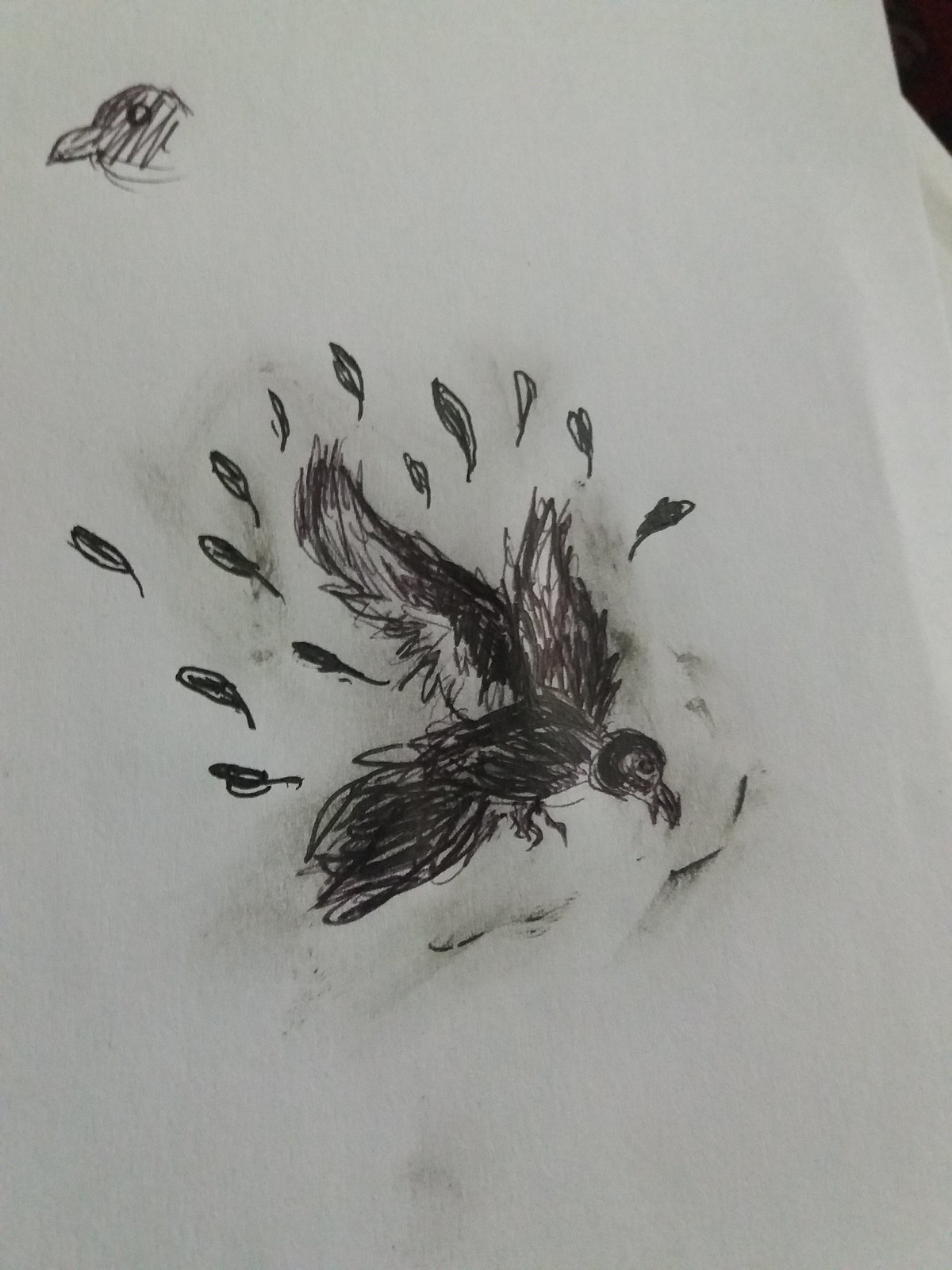A detailed pencil sketch is centrally featured on a white sheet of paper, which is positioned at a slight angle to the left. The edge of the paper is visible at the top-right corner, anchoring the scene. The main subject of the sketch is a bird, captured in a dynamic pose with its head bowed and wings lifted, as if in mid-flap. Intricately drawn individual feathers surround the bird, giving the impression that it is shedding feathers while in flight. The bird is shaded meticulously with pencil, exhibiting various smudges and corrections where parts were erased and redrawn. In the upper-left corner of the paper, there is a smaller doodle of a bird's head, filled in with whimsical squiggly lines, adding a playful contrast to the detailed main sketch.